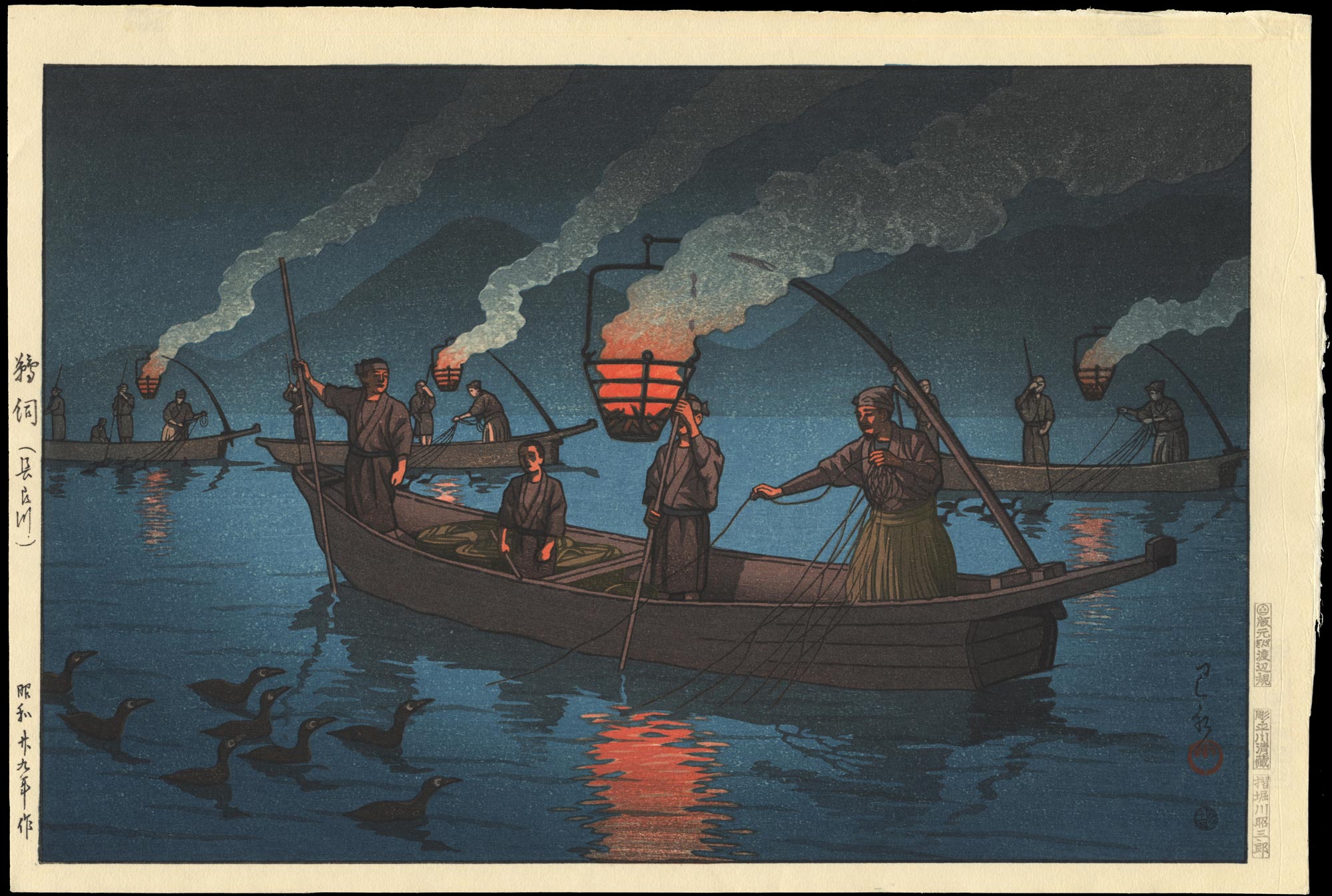In this detailed depiction, the artwork reflects an old Japanese woodcut painting style, reminiscent of the famous "The Great Wave off Kanagawa." The scene features four long, wooden fishing boats populated by fishermen, typically three or four men per boat. Each boat is equipped with large rods reminiscent of Venetian gondolas and nets cast into the water. Prominently, at the bow of each boat, poles extend outwards holding fiery lanterns that produce trailing smoke, likely used to illuminate their nocturnal activity and attract fish.

The setting appears to be either late evening or early morning, inferred from the use of deep, dark blue hues dominating the composition. The scene is enriched by the presence of numerous birds in the bottom left corner, appearing to aid the fishermen by diving for fish. In the background, distant grayish-blue mountains fade into the twilight.

This painting is bordered irregularly with a white edge and traditional Japanese script adorning the left margin, adding to its authenticity. The overall impression is more sketch-like than realistic, capturing a historic fishing method against a serene, yet intricate backdrop.